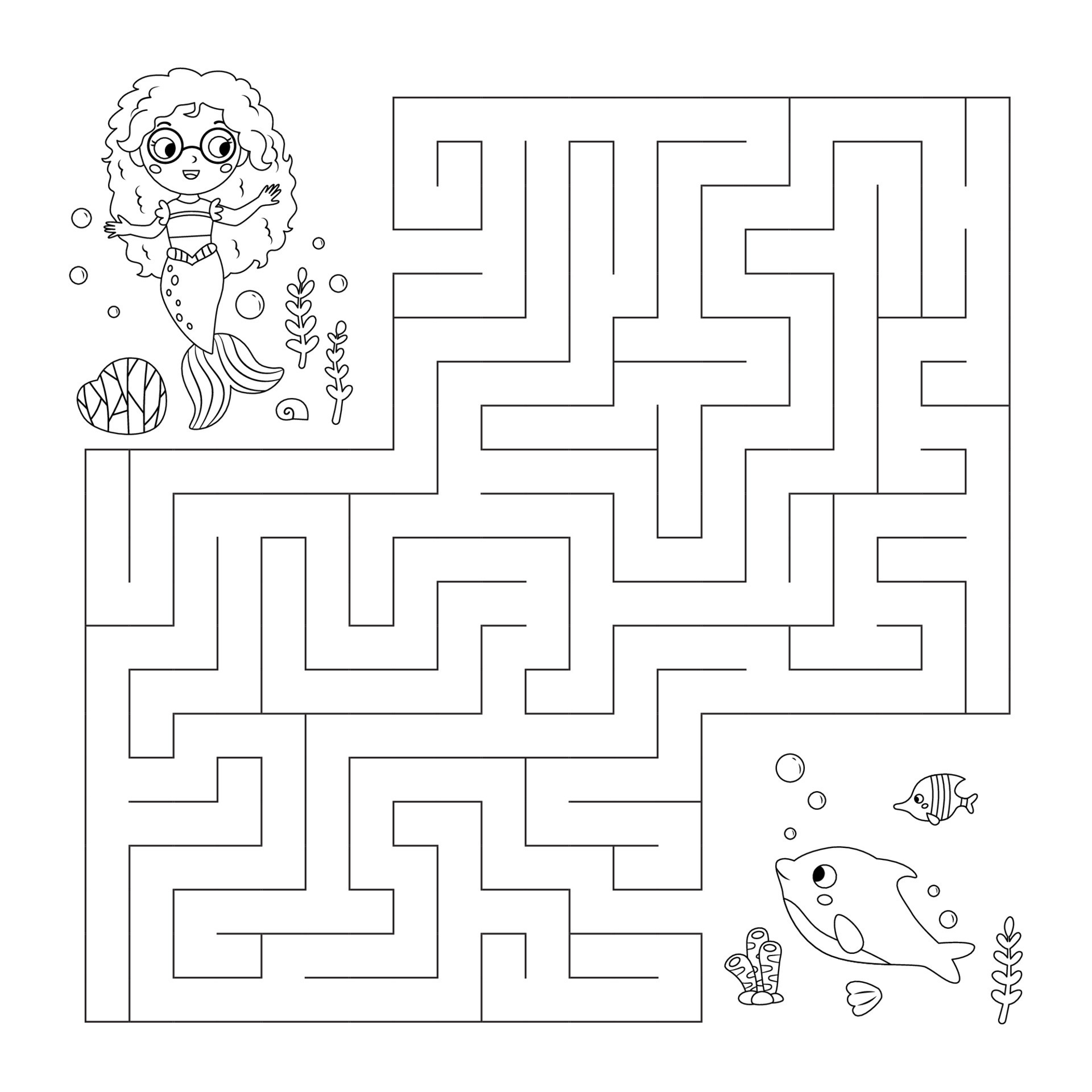The image is a simple, black-and-white maze designed for very young children, perhaps aged four to six, making it ideal for a children's book or a puzzle book. The maze, which covers the entire page, features a mermaid at one end and a fish at the other. The mermaid, who looks about eight years old, wears round glasses, has big curly hair, and is smiling with her mouth open. Surrounding her are bubbles, two small kelp plants, a large seashell, and a smaller shell below her fishtail. She seems to be looking at the puzzle. On the other end of the maze is a fish among bubbles, other sea plants, coral, and a tiny fish floating above a piece of sea kelp. The path through the maze includes multiple dead ends and one correct route, making it a typical maze puzzle where you navigate from the mermaid to the fish or vice versa.